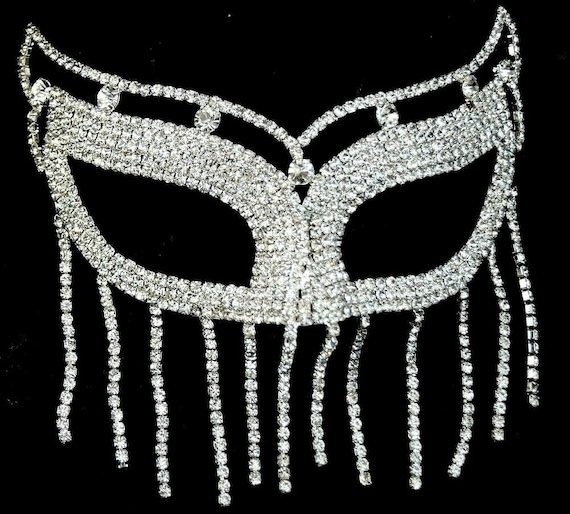The image depicts an intricate jeweled mask set against a solid black background, dominating the entire frame. This mask, reminiscent of those worn at a masquerade ball, is intricately designed with clear, sparkling gemstones, likely cubic zirconia, suggesting a luxurious feel. The mask features a cat-eye shape, with two pointy eye holes and an additional line of gems positioned above the main mask, separated by five larger stones creating a negative space. From the bottom of the eye area, twelve delicate strands of linked gemstones dangle down, somewhat resembling a belly dancer's mask. The composition showcases the gemstone tassels cascading down, while the nose and mouth areas remain mostly uncovered. The photograph, devoid of any text or additional objects, emphasizes the elegance and detailed craftsmanship of the mask, which appears almost surreal or computer-generated in its pristine presentation.